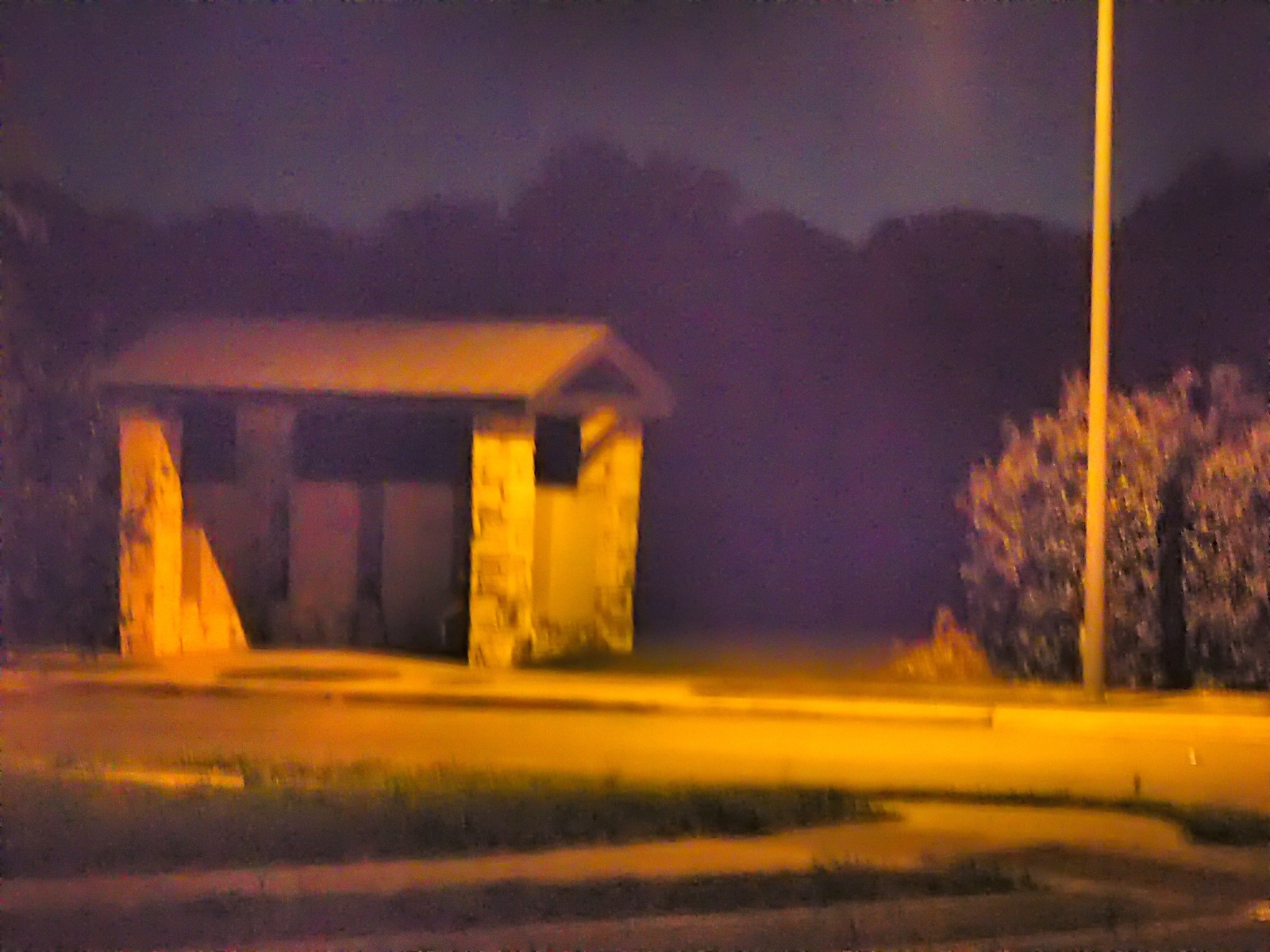This color photograph, slightly rectangular and horizontal, captures a nighttime scene featuring a small stone structure that resembles a bus stop shelter. The structure, with missing windows and a small pitched roof, is illuminated by a streetlight on the right-hand side of the frame, casting a warm yellow glow over the scene. This lighting creates an amber-colored reflection on the concrete pavement in the immediate foreground, where a patch of green grass is also visible.

In the background, a blurry dark blue sky and indistinct, silhouette-like trees add to the overall eerie and somewhat fuzzy quality of the image. Behind the streetlight, a large bush is partially visible. The sky, though dark, still retains some brightness, contributing to the photograph’s slightly surreal ambience. The composition includes a small road in front of the stone structure, and there is no text present in the photo.